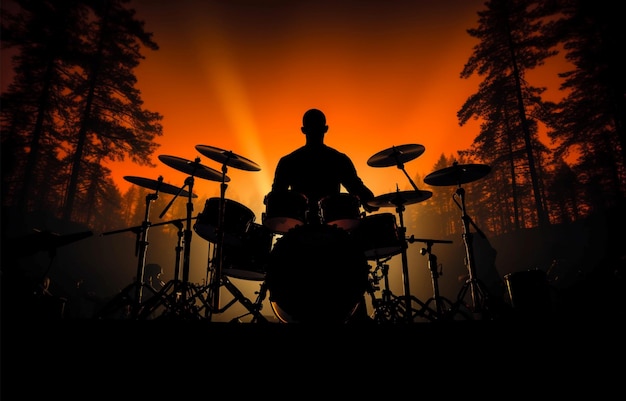The image captures the silhouette of a drummer on a stage or elevated platform, set against the vibrant backdrop of a sunset. The stunning sky features a gradient from dark shades at the top to a fiery orange and finally into a bright yellow where the sun would be. Surrounding the scene are tall trees, likely pine or evergreens, framing the sides of the image. The drummer, potentially a bald or near-bald man, sits centered in the composition, with the drum set silhouetted in black. His left hand rests on a cymbal, and no drumsticks or active drumming motion is evident. The bottom part of the image is completely black, emphasizing the contrast between the silhouette and the luminous sunset backdrop.